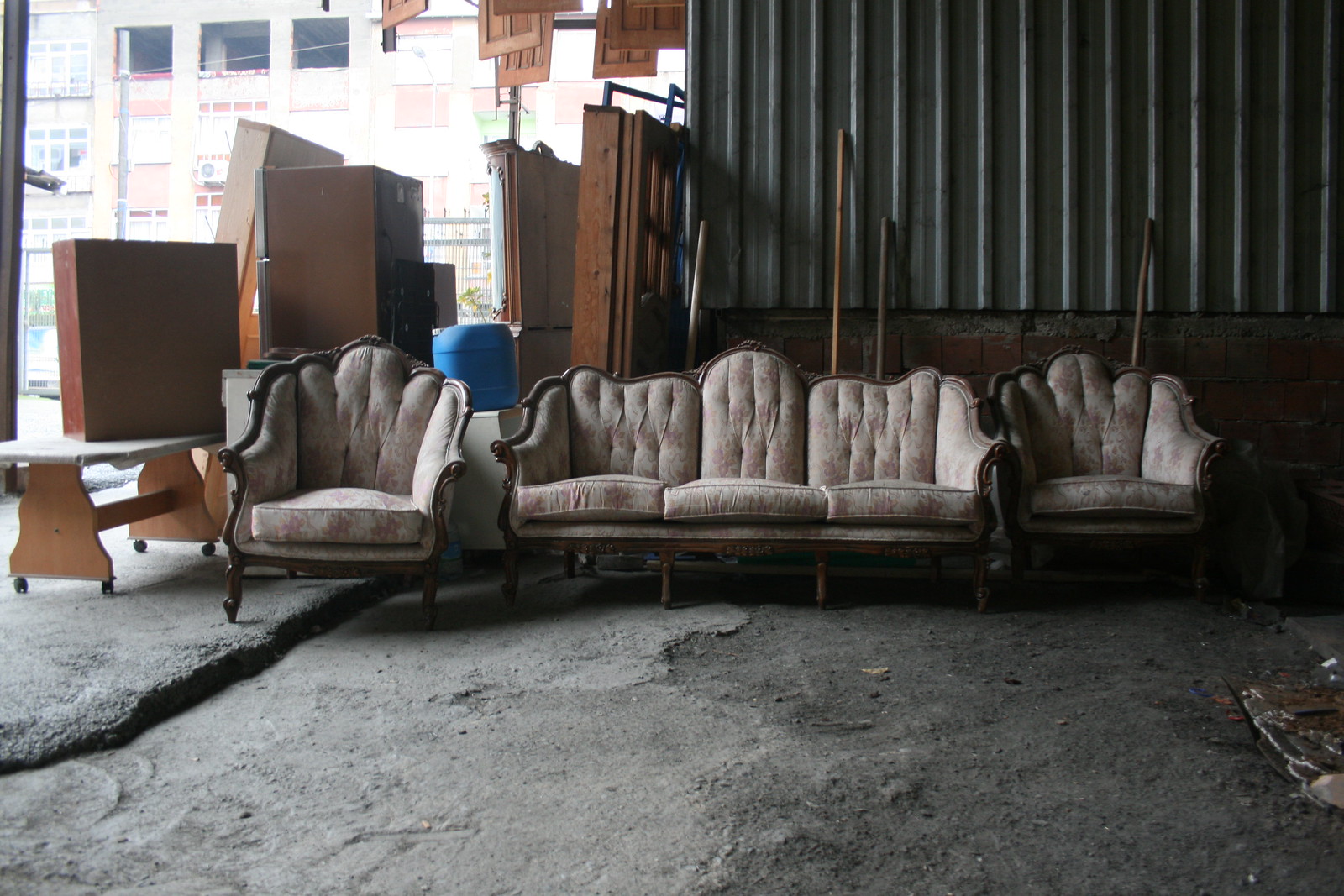This color photograph captures the interior of a run-down storage unit or garage warehouse. The rough gray concrete floor leads up to a back wall made of bricks at the bottom and tin or metal on top. Against this wall is a Victorian-era style seating arrangement, consisting of a large sofa flanked by two matching armchairs. The furniture, though aged and in a state of disrepair, hints at past grandeur with its whitish-beige upholstery and dark wood frames, now dulled to a whitish-brown. In the background, there's a mix of cabinetry, some unattached doors, and a wooden table on wheels, all contributing to the cluttered ambiance. A large window allows some daylight to stream in, revealing the rough-hewn nature of the space and highlighting the antique yet weary charm of the setting.